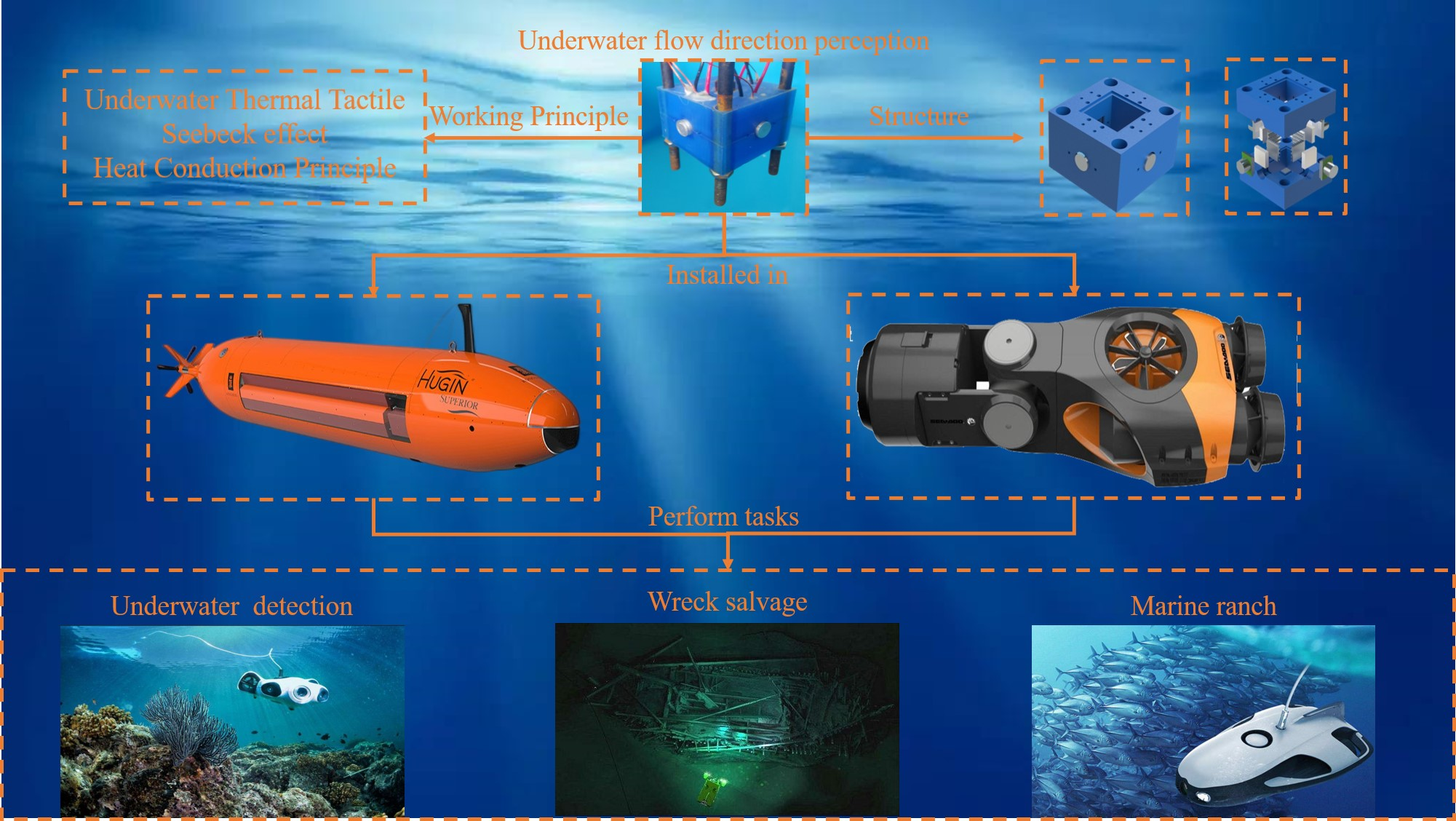This detailed diagram illustrates the principles of Underwater Flow Direction Perception, focusing on the Underwater Thermal Tactile Seebeck Effect and Heat Conduction Principle. The visual layout highlights an array of underwater vehicles, such as submarines and semi-submersible units, which perform various tasks including wreck salvage, marine ranching, and underwater detection. Key components displayed include remote control mechanisms, internal structures of submarines, and diverse apparatuses crucial for these operations. The diagram delves into the working principles and construction details, showing screws, connecting devices, and fastening mechanisms for mounting components. The color scheme features bright blues, oranges, and blacks, evoking an oceanic setting at various depths. There are multiple images depicting these machines in action across different underwater environments, underscoring their installation and operational capabilities. Text labels provide further explanation, detailing underwater flow detection, thermal tactile effects, and essential working principles essential for these marine activities.